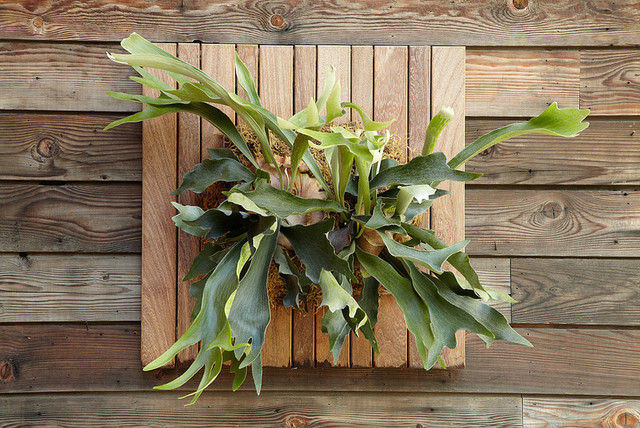This image features a vibrant, green tropical plant with a trunk and roots emerging from some dry material, possibly straw. The plant boasts an array of leaves in various shades of green, extending in all directions, and resembling the shape of a dog’s paw. It is placed on a wooden stand composed of horizontal and vertical wood planks, reminiscent of an 8x8 picture frame, all exhibiting a blend of dark and light brown hues with a pronounced wood grain. The entire setup rests on a larger wooden deck or countertop, with a background of vertical wooden slats arranged in a rough, rustic pattern. This artistic composition, photographed from a top-down perspective, appears to be an outdoor scene designed to highlight the natural interplay between the living plant and the earthy wood elements.